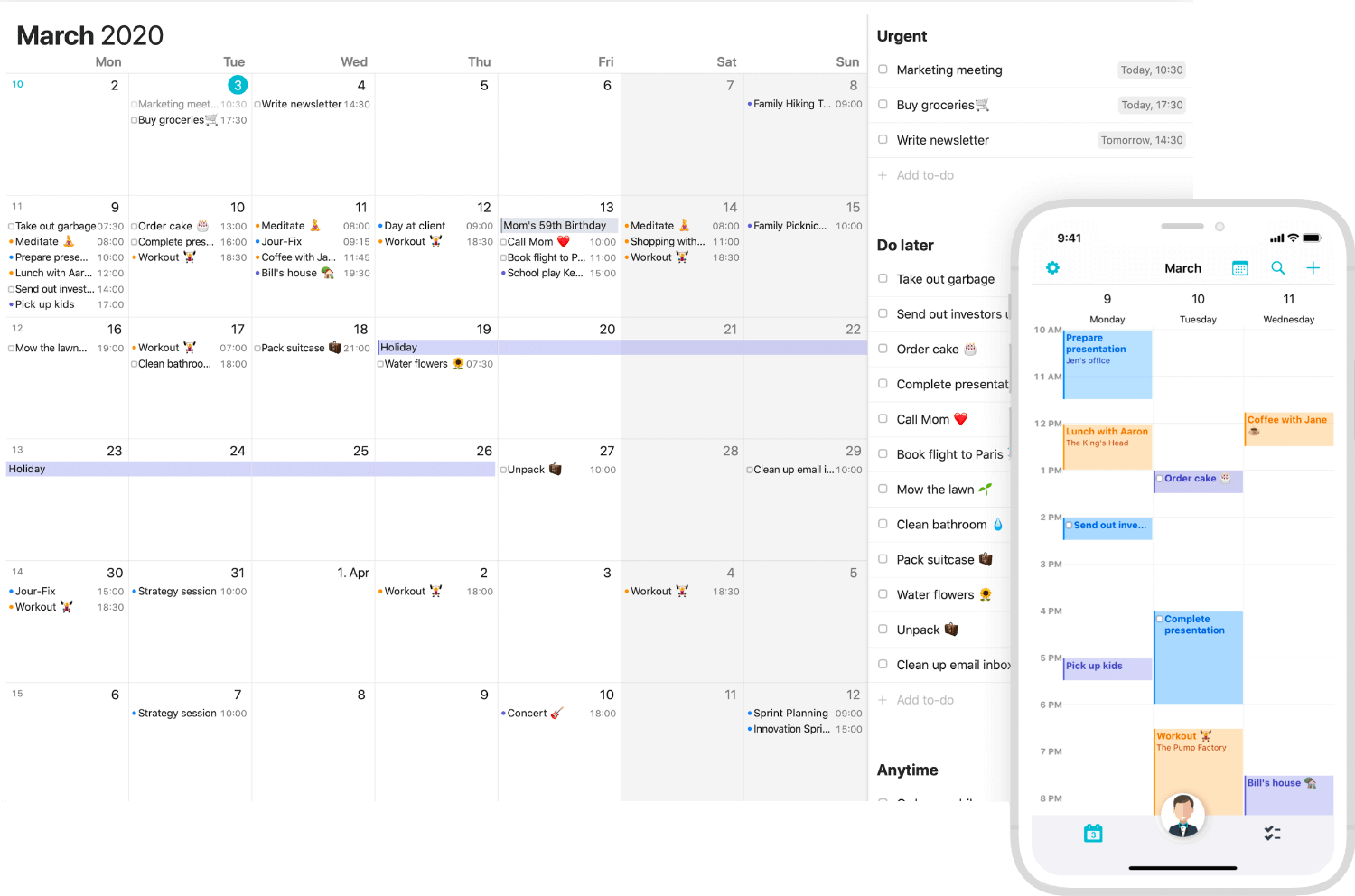The image features a detailed calendar for March 2020, marked with various personal and professional entries. On certain days, specific events and reminders are noted, such as "Mum's 59th Birthday," "Day at Client," "Workout," "Water," and "Flour," indicating a blend of personal plans and household tasks spread across the month. Adjacent to the calendar, on the right side, is a categorized to-do list. This list is divided into sections based on urgency: 

- **Urgent:** Tasks like "Marketing Meeting," "Buy Groceries," and "Write Newsletter."
- **Due Later:** Errands such as "Take Out Garbage," "Order Cake," and "Call Mum."
- **Any Time:** Tasks under this category are not visible in the screenshot.

The far-right side of the image reveals a screenshot of a mobile phone displaying what appears to be a mobile version of the same app. This app version employs a color-coded panel system to organize daily entries, showing only three days at a time side by side, with the option to scroll for more information. This mobile interface allows for quick and organized access to one's schedule and tasks on the go.